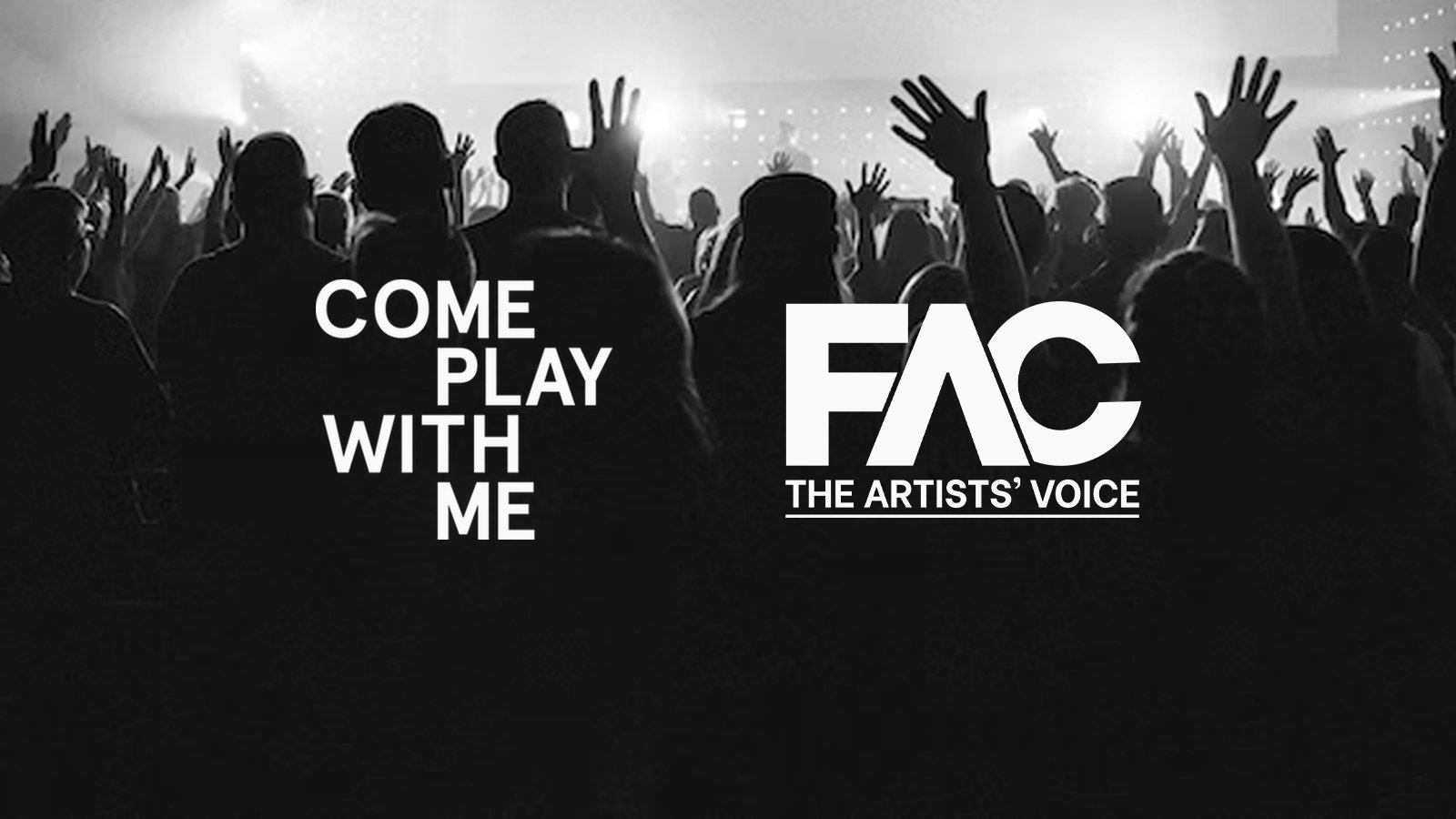The black and white image appears to be an advertisement or poster for a concert or performance. It captures the backs of at least 50 people, their heads silhouetted against the dark background. Most individuals have their hands raised, suggesting a lively and engaging atmosphere. Far in the distance, a performer stands on stage, illuminated by bright lights. To the left of the image, bold white capital letters spell out "Come Play With Me," while to the right, "FAC" is prominently displayed above "The Artist's Voice," both underlined. This suggests a promotion of local venues for concerts and similar entertainment.